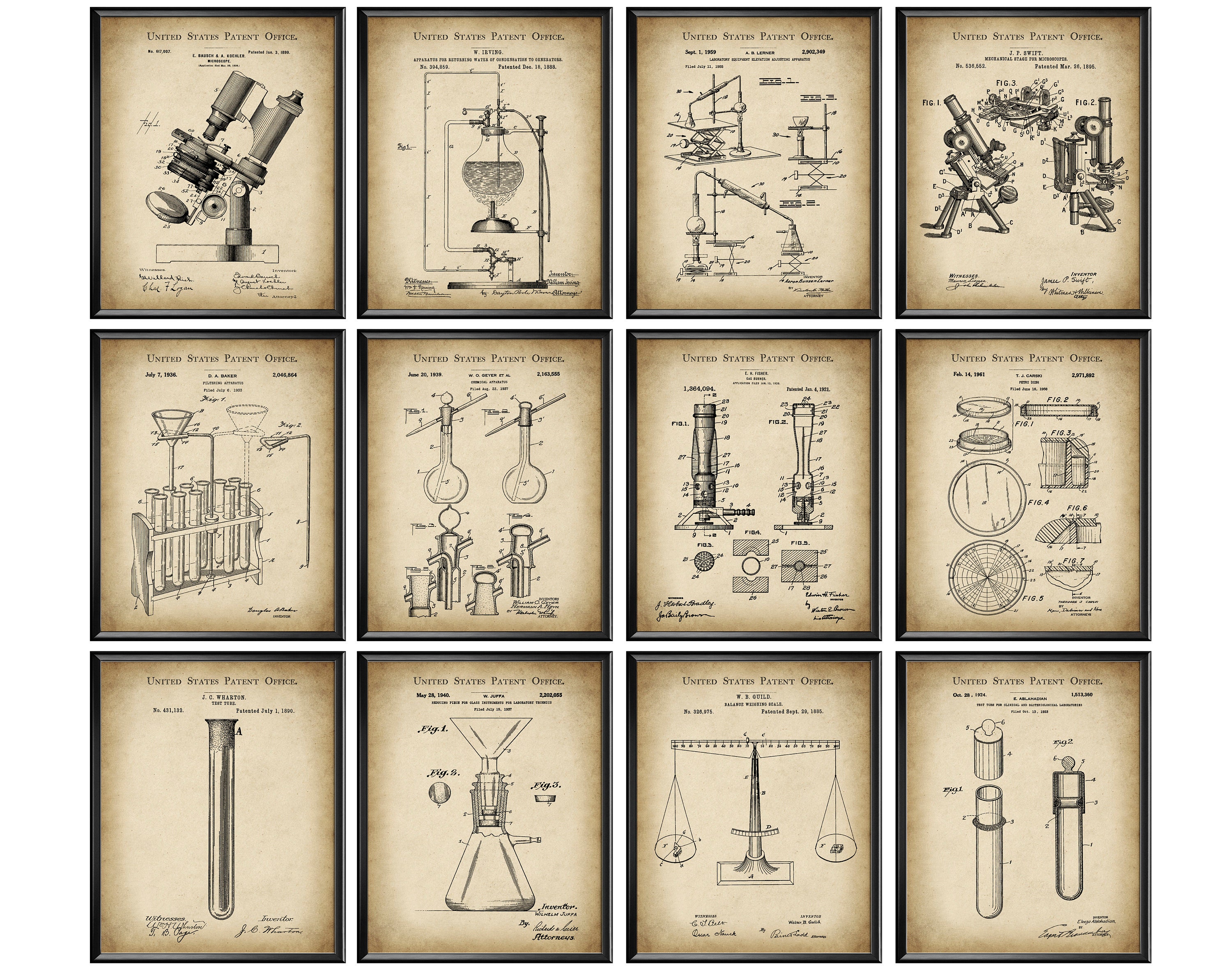This image features a detailed arrangement of aged, light yellowish-brown papers displayed in twelve black frames, organized in three rows and four columns. Each paper is titled "United States Patent Office" at the top, indicating that these are patent illustrations. The papers appear old, with a beige color that's lighter in the middle and darker around the edges. The top-left frame showcases a schematic of a microscope, while the top-right corner features a telescope angled towards the lower left. The middle row appears to focus on various scientific apparatus, including numerous beakers, tubes, and funnels. The bottom row continues with more illustrations of scientific equipment, including glass tubes and a balance scale. This collection of framed art prints offers a fascinating glimpse into historical patent diagrams primarily highlighting scientific instruments and gadgets.